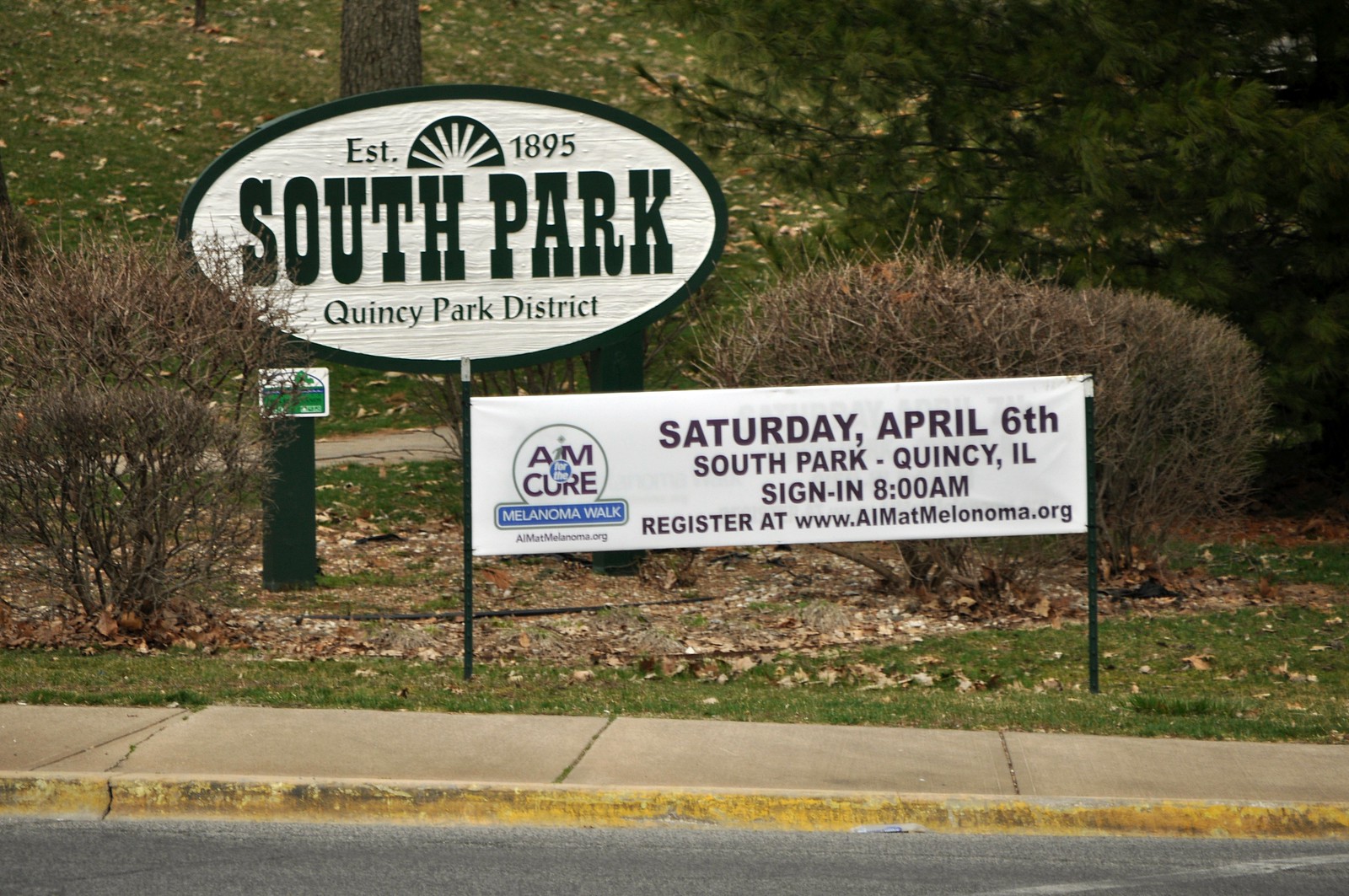This detailed photo captures two adjacent signs standing side-by-side in a park setting. The primary sign, a large oval one, prominently displays "South Park" in big font, with "Established 1895" and "Quincy Park District" written above and below respectively. A green-and-white color scheme, complete with a small sun logo above, is featured on the sign, which stands on green posts in a grassy area. 

Beside it, another rectangular banner announces an upcoming Melanoma Walk event: "Aim to Cure Melanoma Walk" on "Saturday, April 6th, South Park, Quincy, Illinois" with a sign-in time of "8 a.m." and a registration link to "www.aimattmelanoma.org." The banner, also in green-and-white, is mounted on green metal poles.

The surroundings indicate an early spring or late fall setting, characterized by bare shrubs, fallen leaves scattered across a green hill, and a mix of trees including a large pine. A paved asphalt street and a sidewalk with a yellow curb run parallel to this grassy expanse, adding structure to the scene. The color palette is vivid with whites, greens, tans, blacks, and yellows seamlessly integrated into the park's landscape.